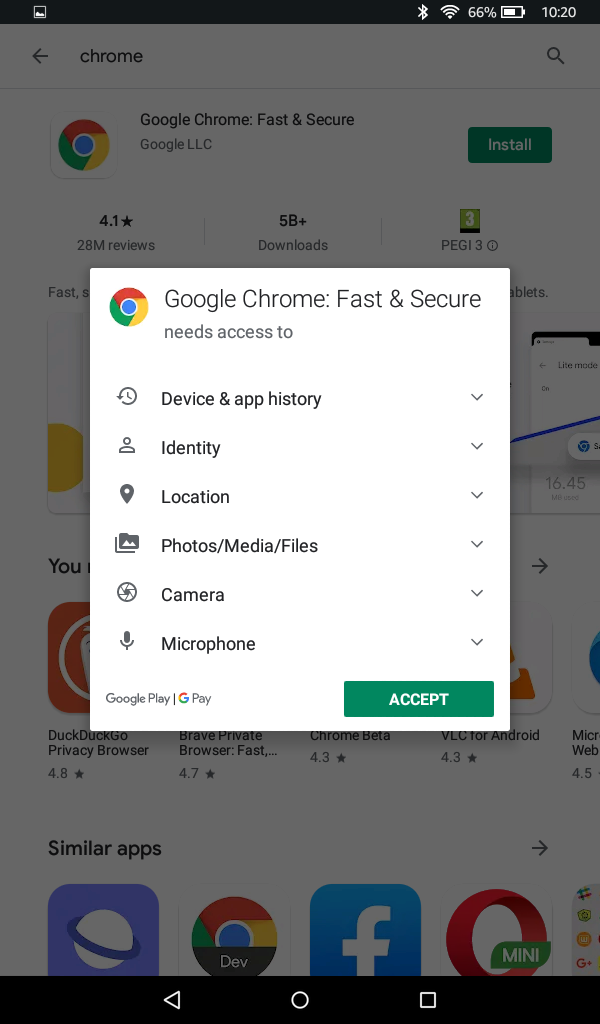The image depicts a Google Chrome installation prompt on an Android device. The top section showcases a white overlay page displaying the Google Chrome logo along with the title "Google Chrome: Fast & Secure." Below this, there's text indicating that Google Chrome needs access to various device features, including:

- Timer, Device, and App History (with a dropdown arrow)
- Identity (with a dropdown arrow)
- Location (with a dropdown arrow)
- Files, Photos, Media (with a dropdown arrow)
- Camera (represented by a circle with a black dot in the middle and accompanied by a dropdown arrow)
- Microphone (with a dropdown arrow)

A green "Accept" button with white lettering is positioned towards the bottom of this overlay. Below this button, there's a note saying "Google Play / GPay."

Beneath the overlay, the screen shows:
- Battery percentage at 66%
- Current time as 10:20
- A Chrome icon alongside a back arrow and a magnifying glass (search icon) to the right.

Immediately under this, the larger page in the background features:
- The Google Chrome logo with the title "Google Chrome: Fast & Secure" by Google LLC.
- An "Install" button.
- Star rating of 4.1 based on 28 million reviews.
- Information on 5 billion downloads.
- A certain level indicated by "3 regedit 3."

Below this, the screen briefly reveals icons for various other apps.